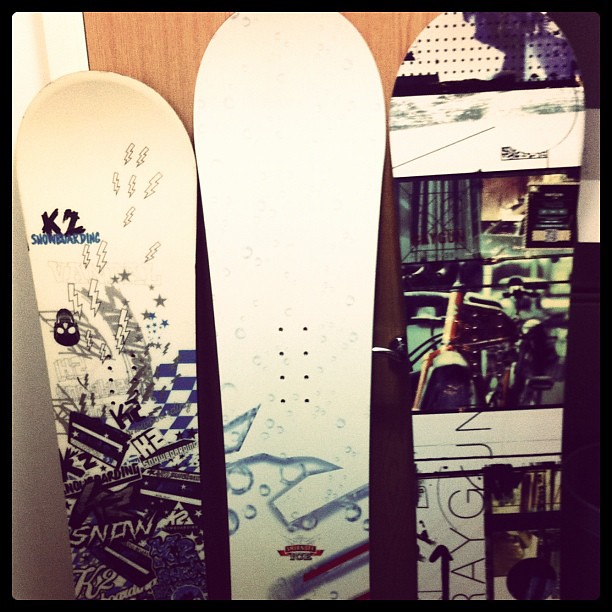This photograph, with a vintage black border suggesting it's from the '90s, captures three skateboards propped against a brown wooden door, with a white wall seen on the left side. Each skateboard is devoid of wheels and bindings, focusing the attention entirely on their intricate designs. The skateboard on the left is white, adorned with a variety of graphical elements, including an upside-down skull and black and blue designs that resemble lightning bolts. The middle skateboard, also white, features a simplistic design with black dots arranged in a line and a blue pattern at the bottom, possibly resembling water droplets. The skateboard on the right showcases an eclectic mix of black and white graphics, including a depiction of a white tower, a series of everyday objects like books, and abstract patterns. All three skateboards highlight a blend of industrial and artistic themes, creating a visually striking display.